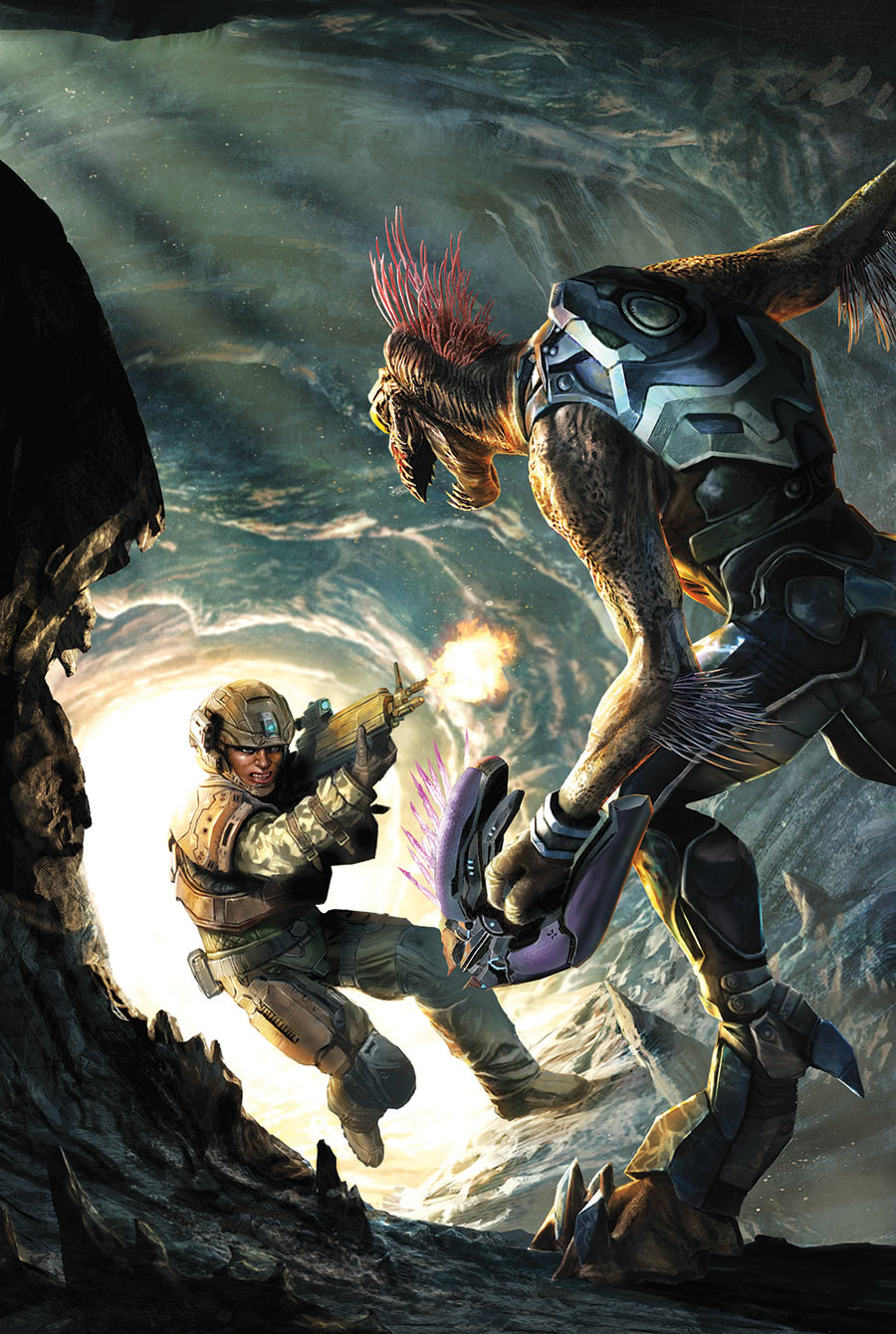In this detailed hand-drawn and colored illustration of a scene from Halo, a formidable alien warrior commands attention in the foreground. The alien, wielding the infamous spike gun in its left arm, is clad in menacing, metal carapace-like armor that protects its torso and legs but leaves its muscular arms exposed. Its right arm dramatically extends off the screen, seemingly about to hurl an unseen object at the human adversary. This creature's menacing visage is accentuated by a fierce, red mohawk-like crest, an open mouth showcasing razor-sharp teeth, and glaring yellow eyes. Its posture, with a large foot sporting a rear talon, exudes raw power and aggression. Feathered protrusions emerge from its elbows, adding an eerie grace to its terrifying appearance.

In stark contrast, a lone soldier is positioned in the background, facing towards us. He is caught mid-stride, balanced on his left leg with his right leg bent at a 90-degree angle, poised to advance. The soldier is depicted in full combat gear, with an army uniform and a helmet that features a distinct blue LED light in the center. He aims his rifle with a steely focus, the weapon discharging a burst of fire towards the alien. 

The scene unfolds within a dimly lit tunnel, its atmosphere further defined by small stalagmites sprouting from the ground and a few stalactites hanging precariously from the ceiling. A bright, almost blinding light spills into the tunnel from behind the soldier, casting his silhouette into dramatic relief as he steps from the outside world into the confined, claustrophobic space of the tunnel. The composition captures a moment of intense conflict and imminent danger, blending the raw fury of the alien with the determined resolve of the human soldier.